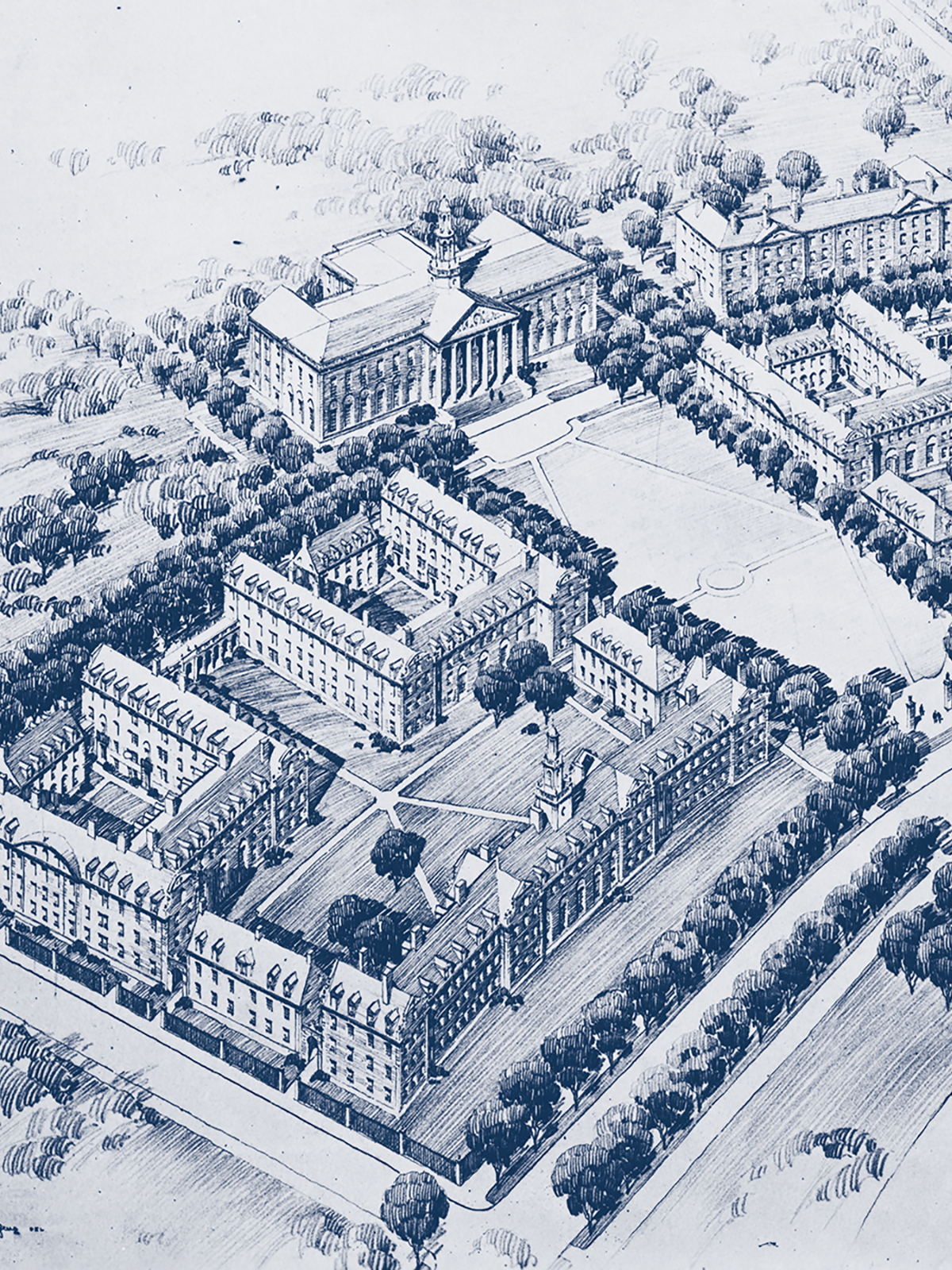This detailed, pencil or pen-styled black and white drawing is an aerial view of a regal, government-type complex. At the center is a large, grand building reminiscent of the White House, characterized by its prominent columns and well-manicured lawn. Surrounding this central building are multiple four-story structures, organized in a grid that resembles city blocks. Trees are planted in neat, square patterns around the buildings, adding to the structured and elegant appearance of the area. The image feels like a blend of a blueprint and a sketch, with clearly defined buildings filled with windows, courtyards, and what appears to be driveways or sidewalks weaving through the complex. The entire scene is devoid of any skyline, focusing solely on the top-down perspective of this meticulously designed space.